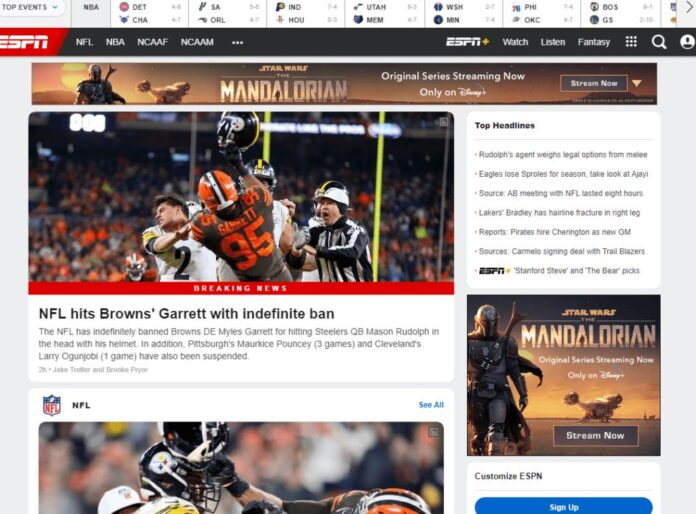**Detailed Caption:**

The screenshot showcases the ESPN website, where the brand's distinctive white "ESPN" logo appears against a red background in the top left corner, albeit partially cut off. Adjacent to it, a black navigation bar extends horizontally, featuring menu options including "NFL," "NBA," "NCAAF," "NCAAM," and a three-dot icon for more options. Towards the right side of this bar, starting from the center, icons and labels include "ESPN+" with a yellow plus sign, "Watch," "Listen," "Fantasy," a grid of nine white dots forming a square symbol for additional tools, a search icon, and a user profile icon.

Just below the navigation bar, there is a promotional banner for the original series "The Mandalorian", streaming exclusively on Disney+. The banner has a brownish color scheme and contains a "Stream Now" button with a dropdown arrow on the right.

Further down, the main content of the page features a photograph depicting football players in action along with a referee, coinciding with a "Breaking News" segment. The headline reads: "NFL indefinitely bans Browns' DE Myles Garrett for hitting Steelers' QB Mason Rudolph in the head with his helmet." Additional details reveal suspensions for other players involved, including Pittsburgh's Maurice Pouncey, who received a three-game ban, and Cleveland's Larry Ogunjobi, who faced a one-game suspension.